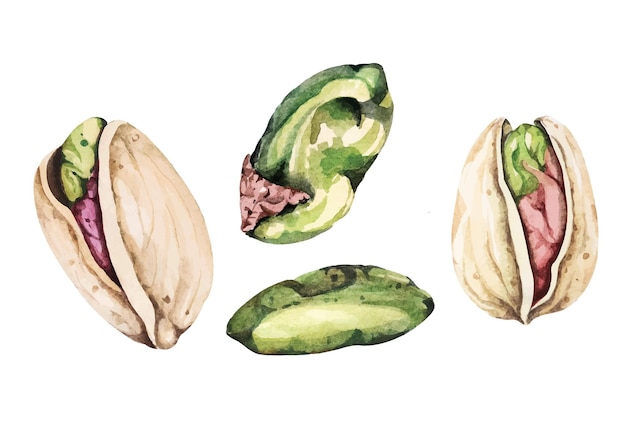This illustrated image, resembling a watercolor painting, depicts various states of pistachios, both in and out of their shells. To the left, a tan-colored pistachio shell is slightly cracked open, revealing a reddish-pink interior with a greenish tip. Adjacent to it, towards the right, are two slightly lumpy, oval-shaped pistachio nuts. The top one is mostly green with a hint of pink on the bottom left, while the one beneath it is entirely green with patches of light, dark, and regular green hues. Further to the right, another pistachio shell is visible, more significantly split open to reveal its colorful contents, showcasing a mix of pink and green tones. The irregular shapes and varied shades emphasize the natural, organic form of the nuts.